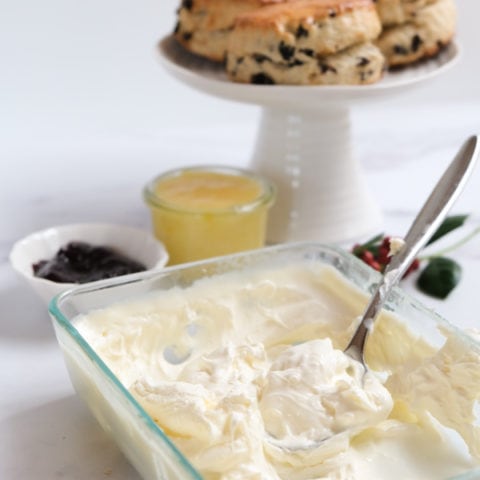The image depicts a serene, white-themed dessert setup. Centrally positioned, a white pedestal holds three scones, potentially blueberry or chocolate. Below the pedestal is a clear container likely filled with lemon curd. Adjacent to the lemon curd sits a small white bowl containing what appears to be blackberry preserves. In the foreground of the image, a rectangular glass dish contains light, fluffy whipped cream, with a silver spoon ready for serving. The overall composition highlights the whipped cream while subtly featuring the scones, lemon curd, and preserves, against a clean white background.